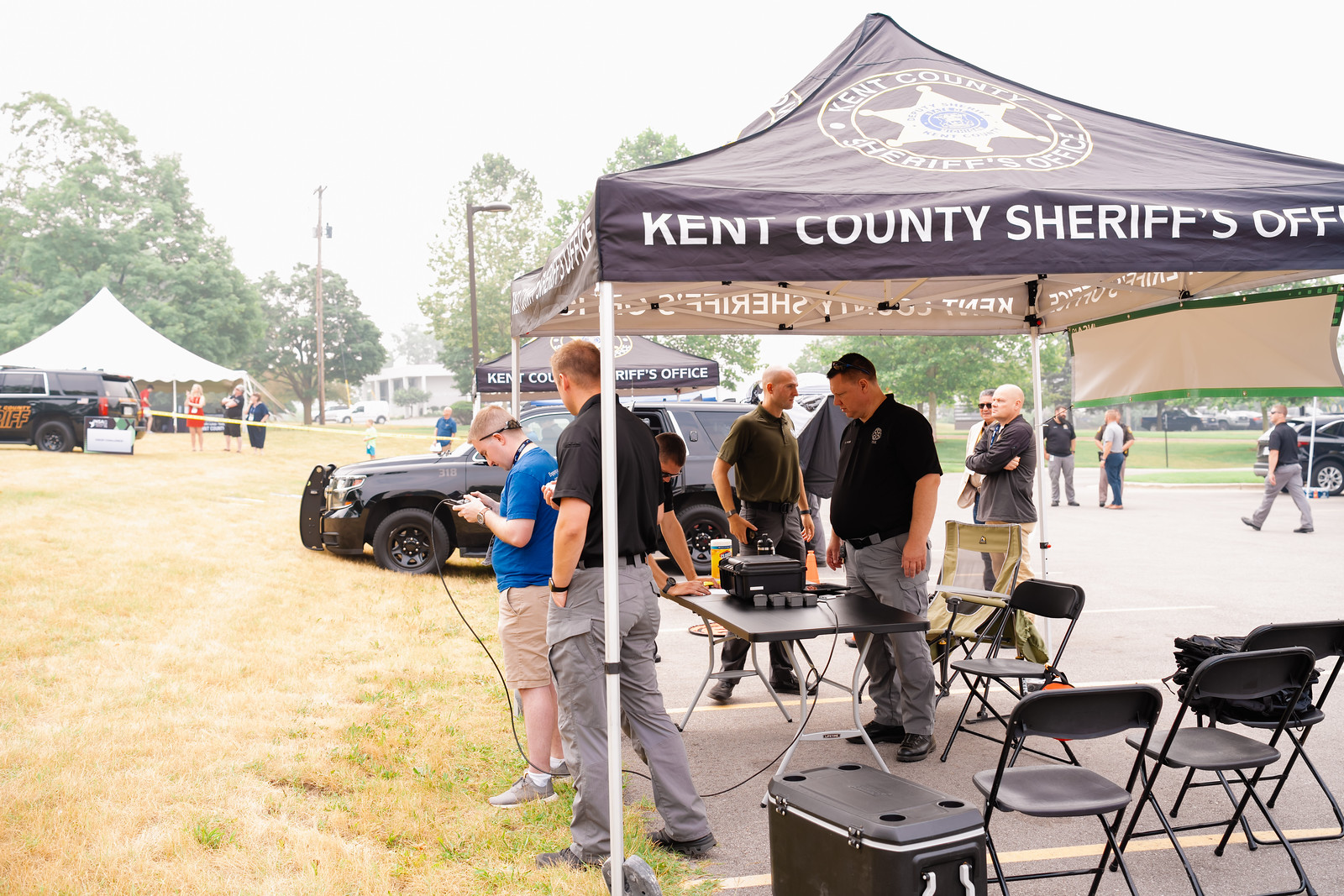The photograph showcases an outdoor group event organized by the Kent County Sheriff’s Office, featuring two black tents, each adorned with the Sheriff’s badge logo and the text "Kent County Sheriff's Office." In the lower right quadrant of the image, the main tent shelters a table with various equipment, eight folding black chairs, and a black cooler. Under this tent, six individuals, including a mix of men in black shirts and gray slacks, and a woman in a blue top and khaki shorts, are engrossed in their devices, paying no attention to one another. Surrounding the tent, the dark gray pavement contrasts with the green grass where the woman stands. In the background, approximately five other people mill about near additional tents and a noticeable black sheriff’s car. The tents are part of a broader setup aimed at possibly advertising or showcasing the Sheriff’s services, with no one seated in the available black folding chairs.